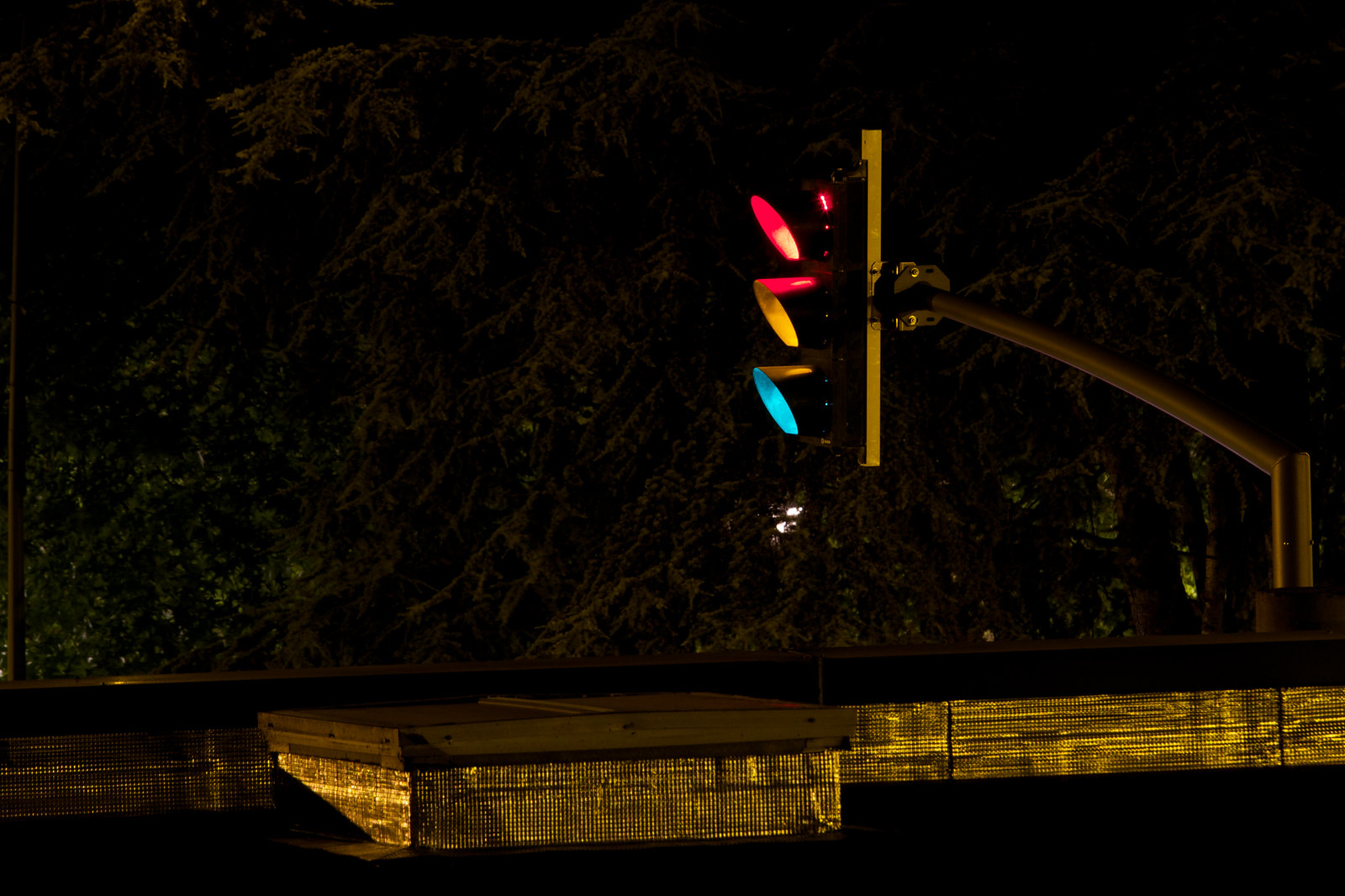The photograph captures a traditional red, yellow, and green traffic light at night, prominently propped up high in the center of the image by a metal pole. The traffic light is vertically aligned, with its pole extending out horizontally to support the signal. Uniquely, all three lights – red, yellow, and green – are illuminated, creating a rare and striking effect against the dark, night backdrop. The scene is set in a dimly lit urban area, with indistinct shapes suggesting possible cityscape elements, including what might be a building or wall at the bottom, and indeterminate dark green trees in the background. The metal infrastructure of the pole reflects light, giving it a silvery or golden appearance. Additionally, a subtle white light peeks through the trees below the traffic light, adding a tiny glimmer to the overall dark ambiance.